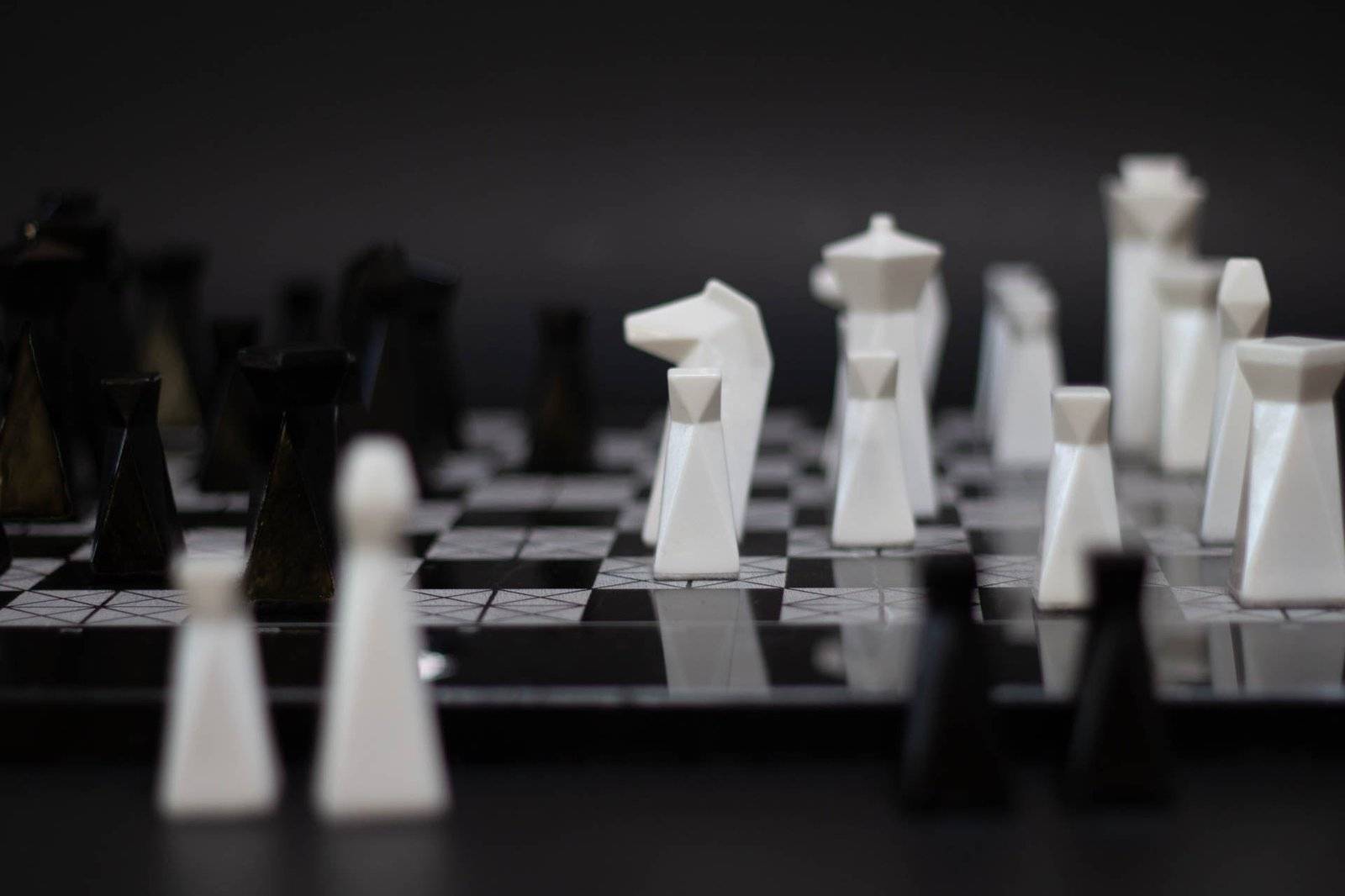The image captures a close-up, landscape-oriented view of a polished and elegant chess set, focusing predominantly on the white pieces. The chessboard features gray and black squares, with the gray squares adorned by thin black cross lines. The shallow depth of field highlights a white piece, likely a rook, standing prominently in the center. This piece is wider at the bottom and ascends straight to a neatly angular peak on a gray square. Surrounding this focal point, the pieces become progressively blurry, creating depth and contrast.

On the right side of the board, mostly white pieces are visible, including a distinct, squared-off knight that resembles a horse's head, partially enveloped in shadow. To the bottom right, there are out-of-focus black pieces. The left side of the image, although less detailed, suggests the presence of black pieces, some of which are slightly intermingled, reflecting a game in progress. Captured white pieces rest off the board in the foreground, further emphasizing the dynamic nature of the setup.

The chessboard and pieces are highlighted by their reflective, well-polished surfaces, implying they may be crafted from plastic, 3D-printed material, or smooth stone. These reflections add a sophisticated touch to the scene. The background, a deep dark gray, brings a subtle and elegant contrast, making this high-end chess set the centerpiece of the photograph.